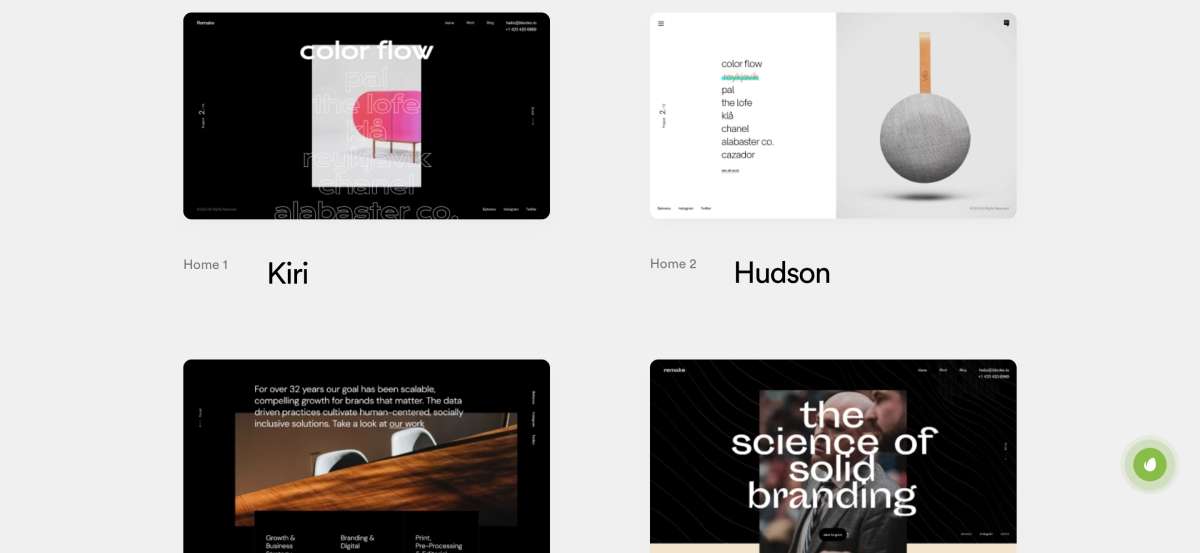The image features a grey background with four distinct boxes arranged in a 2x2 grid. 

In the top-left box, there is a black background with a central grey box containing an oblong, purple object. White text overlays this scene, reading "Color Flow" at the top and "Home 1, Keery" below the grey box.

The top-right box is divided into two sections. The left side has a white area with text that is too small to read, while the right side boasts a grey background with an illustration of a frying pan whose handle is facing upwards. Beneath this is the text "Home 2, Hudson."

In the bottom-left box, a black background showcases a grey and brown terrain-like element. There is white text overlaid, but it is too small to decipher.

The bottom-right box features a black background with an image of a person obscured by white text that reads "The Science of Solid Branding." Adjacent to this, in the bottom-right corner, is a green circle with a halo-like effect around it and a white spot in the center.